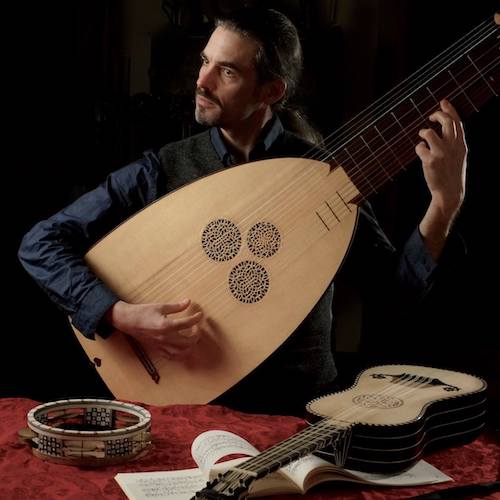In this detailed photograph, a man is prominently featured playing an oversized, mandolin-style guitar with a uniquely wide and flat body, markedly different from a traditional guitar. The instrument has three black, speckled circles on its light wooden base and a dark wooden neck. The man, with long dark brown hair tied in a ponytail, a mustache, and a goatee, is looking intently to his right. He is dressed in a long-sleeved blue shirt paired with a black vest.

In front of him, a red velvety tablecloth covers a table. On this table, a light wood tambourine rests to the left. Nearby is a smaller guitar, also in light wood with a dark brown outer shell, placed atop an open music book with one page slightly folded over. The background of the photograph is dark, emphasizing the man and his instruments as the focal points.